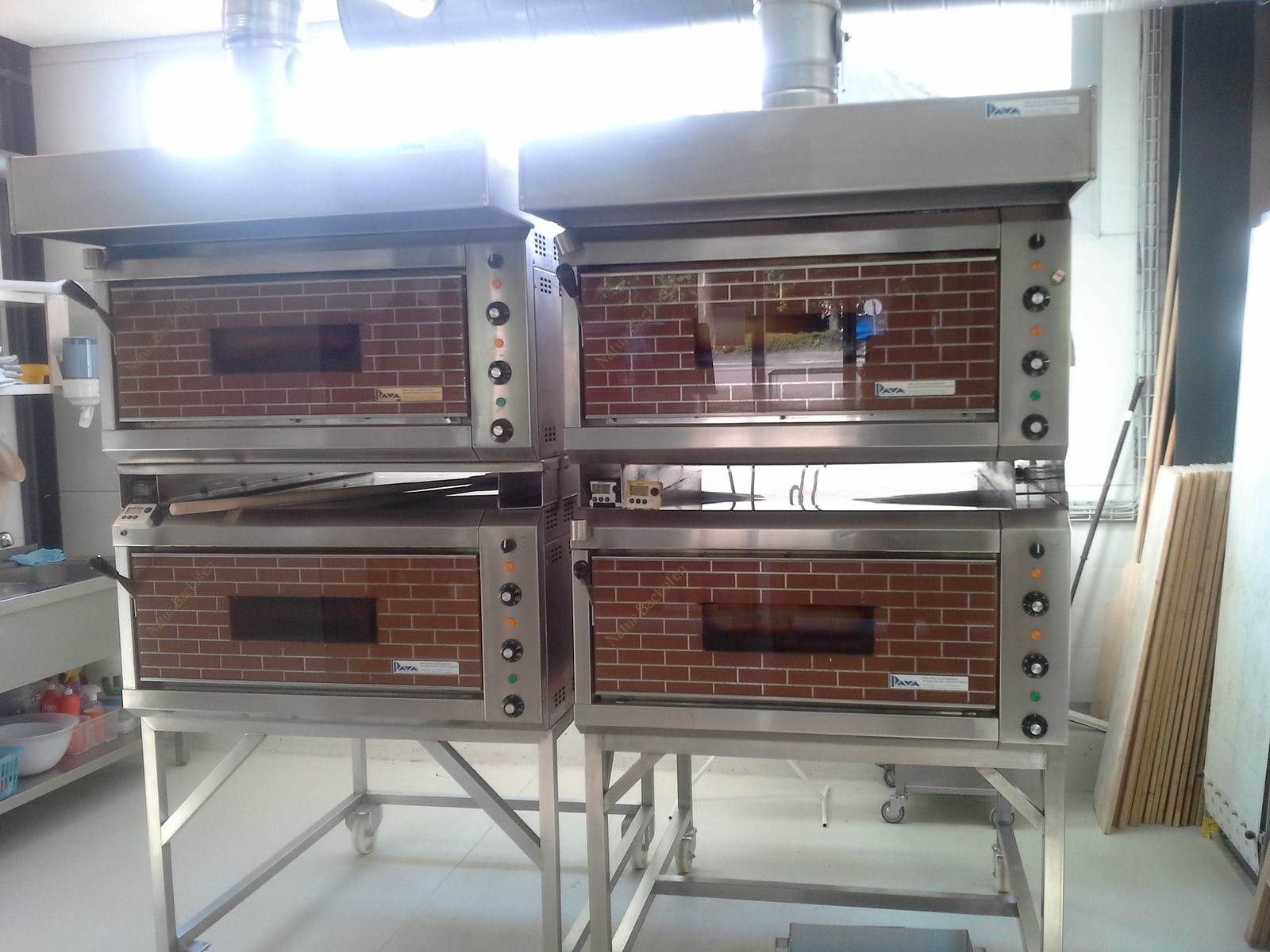The image depicts an industrial kitchen with a distinctive focus on four brick pizza ovens, centrally positioned. Each oven features a silver stainless steel exterior, a brick facade with a rectangular glass door in the middle, and four black knobs on the right side. The ovens are arranged in stacks of two, mounted on metal legs and stands, giving a sturdy, elevated appearance. The backdrop includes large windows that allow intense sunlight to shine through, creating a noticeable glare that slightly washes out the top left of the picture. To the right, some wooden boards are leaning against the wall. The white tiled floor complements the white walls, contributing to a clean, bright atmosphere. On the left side, part of a counter is visible, housing cleaning supplies in a drawer or shelf underneath, along with a large towel dispenser and a sink. The overall ambiance suggests a well-organized, functional kitchen space designed for high-volume cooking.